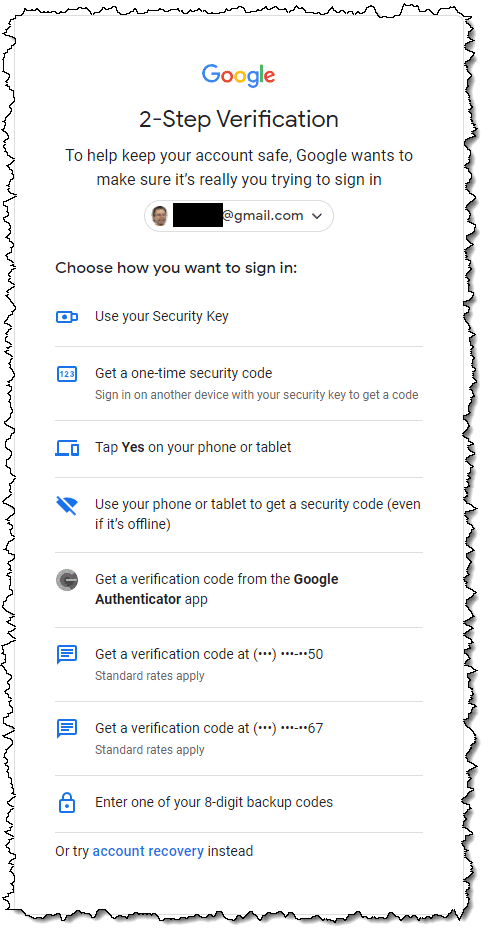This image is a vertical rectangle and features a screenshot of a Google pop-up screen for two-step verification. The entire image is framed by a hand-drawn, squiggly black line that appears to have been made by a pencil, giving it a whimsical and informal touch. The interior of this outlined box has a white background that provides a stark contrast to the detailed content inside.

Centered at the very top of the image is the Google logo. Directly below this, the text "Two-Step Verification" introduces the purpose of the pop-up. A brief explanation follows: "To help keep your account safe, Google wants to make sure it’s really you trying to sign in."

Beneath this explanatory text is an oblong, oval-shaped area containing a blacked-out section of an email address (ending with @gmail.com) and a drop-down arrow, indicating that the user can select different options or accounts.

The section titled "Choose how to sign in" follows, listing several methods with accompanying icons and separated by thin gray lines:

1. **Use Your Security Key**: Represented by a small key icon.
2. **Get a One-Time Security Code**: Sign in another device with your security key to get a code. This option is illustrated with an icon of a numbered box.
3. **Tap Yes on Your Phone or Tablet**: Depicted with an icon showing a screen and a phone layered over it.
4. **Use Your Phone or Tablet to Get a Security Code, Even If It’s Offline**: Indicated by an icon of a Wi-Fi signal with a line through it.

Each method within this pop-up guide is clearly defined with both textual instructions and visual icons, aiding in user navigation and facilitating secure account access.